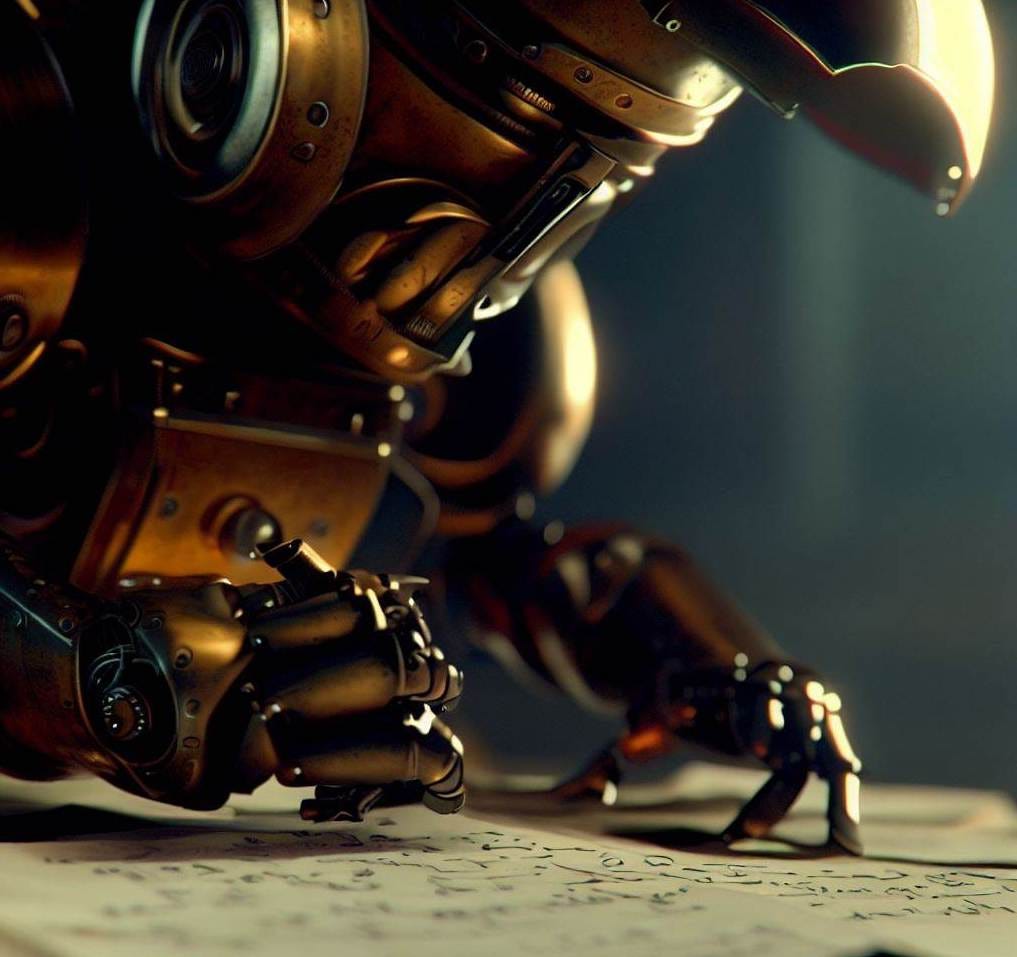The image features a detailed, AI-generated robotic character set against a light, out-of-focus gray background. Occupying the left side of the picture, the robot is meticulously crafted from metal, predominantly in shades of copper and bronze. Its humanoid form includes a large head adorned with a forward-projecting component and a circular section beneath it, resembling futuristic or Pixar-style designs. The robot's right arm, holding a pen, leans over a piece of paper covered in intricate black ink lines, while its left hand stabilizes the sheet. Noteworthy elements include a lens-like ear on the left side of the head, a small square section on the chest, and spider-like, thin metal fingers. Additional details reveal a thin light where the eyes would be, a narrow metallic protrusion suggesting a nose, and a grid-like pattern mimicking a mouth. The robot's actions, leaning in to write or perhaps read on the paper, suggest a scene of meticulous note-taking or drawing.